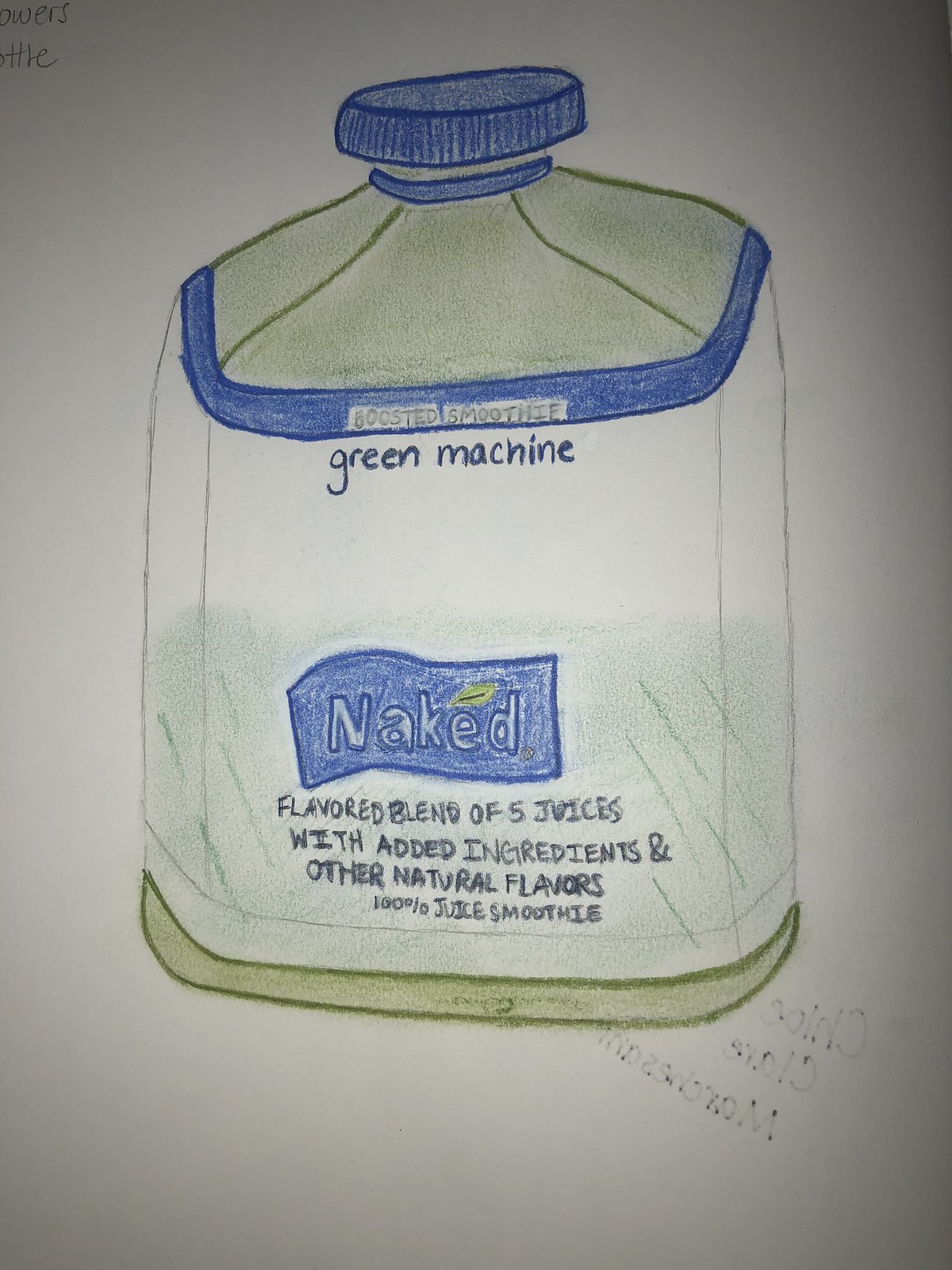This detailed handmade drawing showcases a Naked brand smoothie bottle, meticulously illustrated using either colored pencils or crayons. The beverage depicted is the Green Machine flavor, identifiable by the vibrant green liquid shown within the bottle. The label is accurately rendered, with a white background adorned with blue striping and a blue screw-top lid. The label text clearly states "Naked" as the brand, "Green Machine" as the flavor, and emphasizes it is a "Boosted Smoothie." Further details on the label denote it as a "Flavored blend of five juices with added ingredients and other natural flavors," confirming it as a "100% juice smoothie." The proportions of the bottle in the drawing are slightly taller than the actual product, but overall, the illustration serves as a faithful recreation of the real-world item.